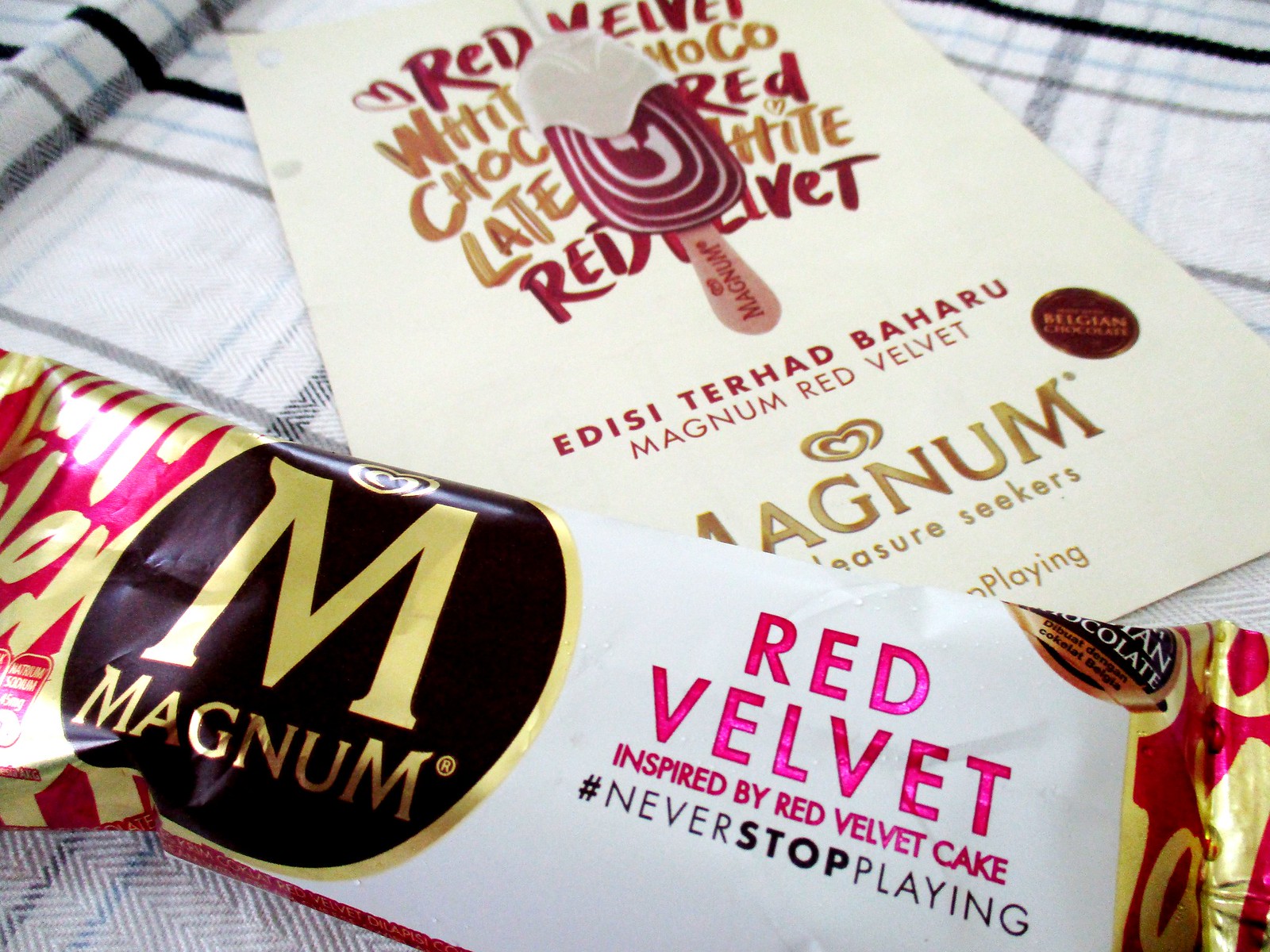The image depicts a Magnum ice cream bar, still inside its wrapper. The wrapper features the iconic Magnum logo, consisting of a black circle with a gold capital "M" and the word "Magnum". To the right of this logo is red text that reads, "red velvet inspired by red velvet cake" followed by a black hashtag, "#neverstopplaying". The wrapper is predominantly a mix of white, gold, black, and pink colors. Additionally, the ice cream bar and wrapper are placed on top of an advertisement card that is laying on a cloth with white, blue, and black stripes. The card itself displays a detailed image of the ice cream bar, illustrating its swirly reddish and white appearance, with a white cream topping. The card features more product information, including the text "Magnum red velvet" and a visual representation showing the white chocolate-covered red velvet ice cream, reinforcing the delicious and enticing look of the treat.